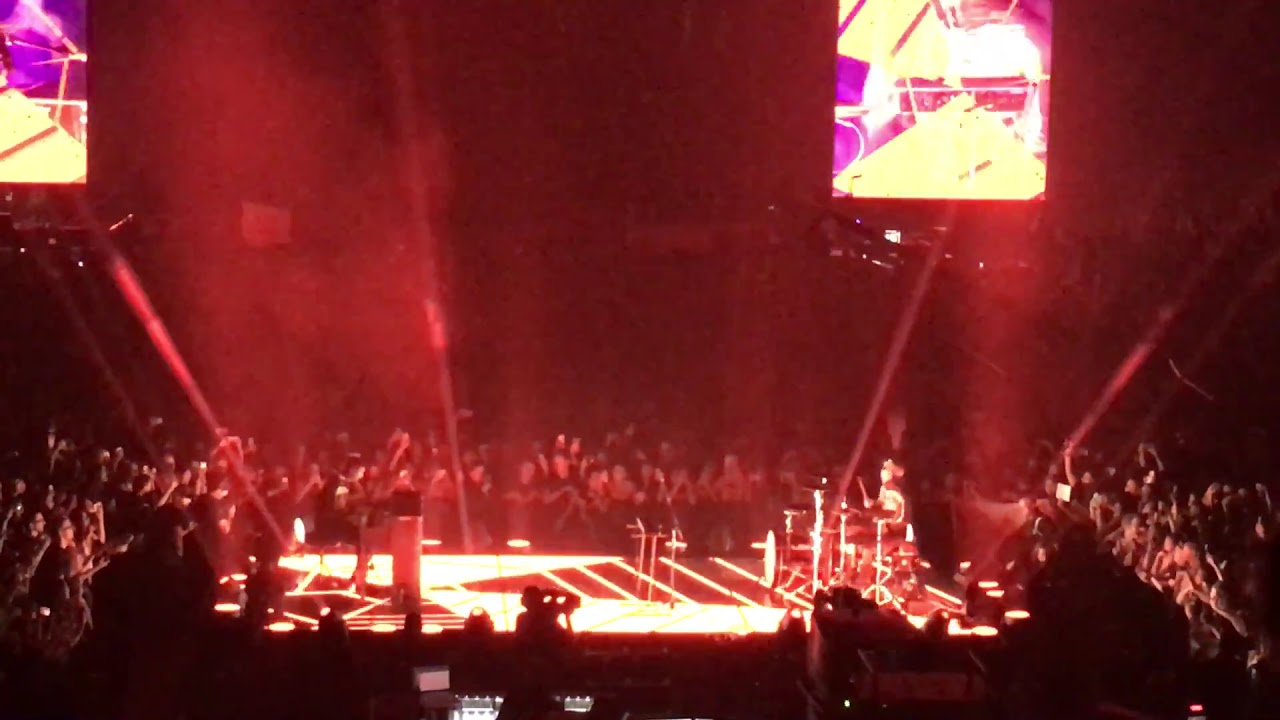The photograph captures the electrifying atmosphere of a large musical concert set in a dark auditorium, with the stage being a central focus illuminated by intense red and orange lighting. Bright, pulsating lights project upward and downward from the stage, casting a vivid reddish hue throughout the venue. The stage, surrounded by a sea of energized fans cheering and raising their arms, is equipped with two prominent screens on either side, likely projecting live footage of the performers to enhance visibility for the vast audience. Amidst the dazzling lights, a drummer with an elaborate drum set can be seen, contributing to the vibrant performance. The details of other performers on stage are less clear, but their presence is felt in the dynamic and immersive visual display.